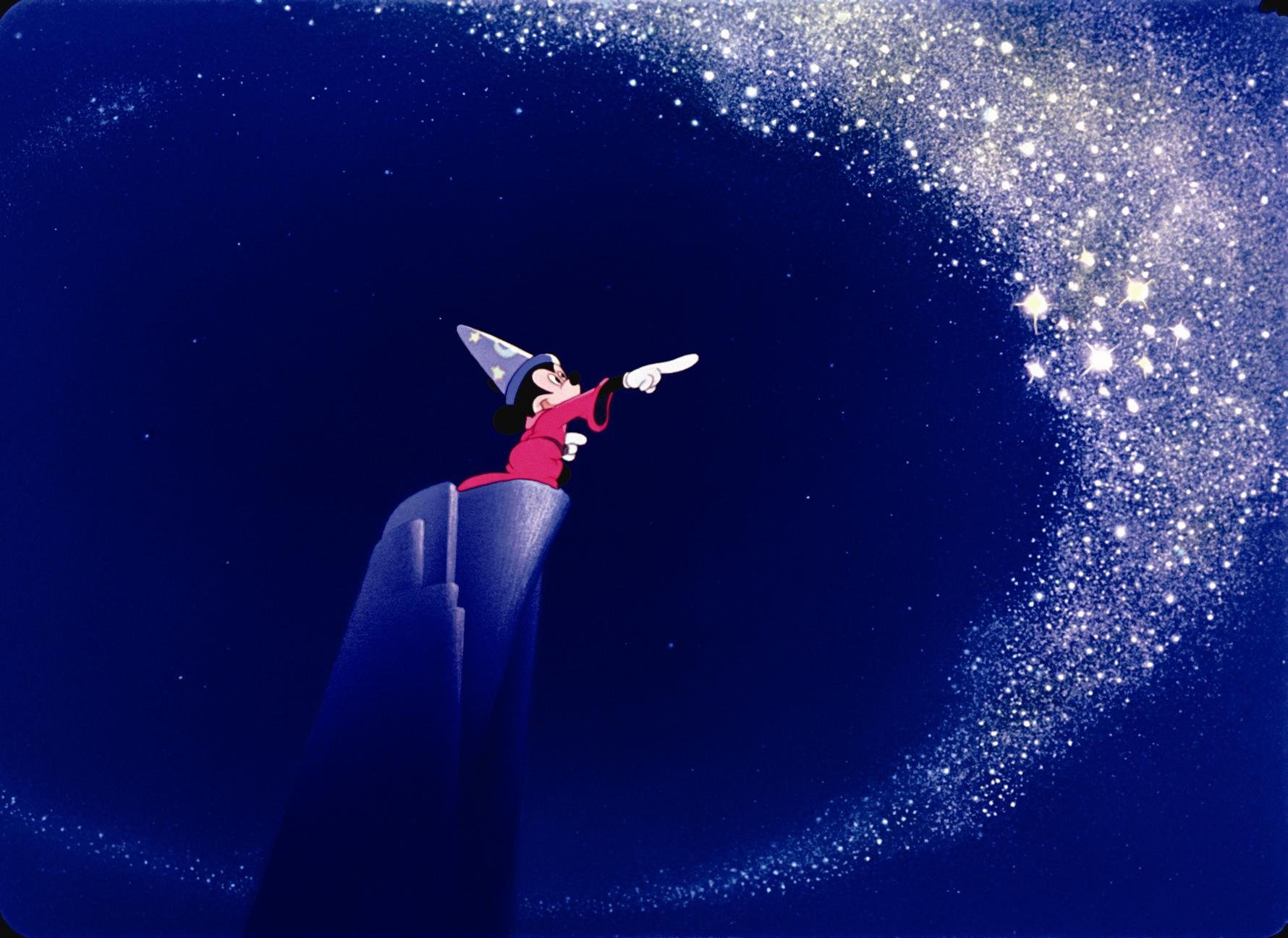In this vivid scene from Disney's "Fantasia," Mickey Mouse is portrayed as a magician, standing majestically atop a natural rock pillar, reminiscent of a small hill. Mickey is adorned in his iconic red robe and wears a blue wizard's hat decorated with stars and a moon. His familiar black ears, light-colored face, and white-gloved hands are distinct, with one of his hands pointing to his right, guiding the viewer's eye towards an enchanting display. In the night sky, a ring of multi-pointed white stars forms a magical circle, appearing to be under Mickey's spell. The sky itself is a mesmerizing blend of varying dark blue shades, with hints of black scattered throughout, enhancing the mystical ambiance of the scene. The landscape and stellar arrangement create a dynamic and captivating visual, showcasing Mickey deep in his wizardly role, conjuring and manipulating the stars in a fantastical display of magic.